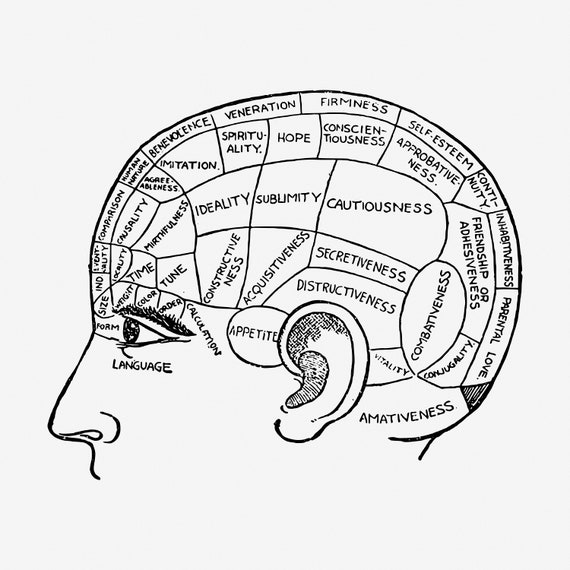This image features a detailed black and white drawing of a human head in side profile, depicted on a very light gray background. The head is illustrated facing left and is cut off just below the nose and ear. The drawing is divided into multiple labeled sections, each representing different areas of the brain. Text is meticulously inscribed within these sections to indicate various concepts, likely related to the study of phrenology.

Starting from the top, notable labels include **Firmness**, **Self-Esteem**, **Inhabitiveness**, **Parental Love**, **Combativeness**, **Mirthfulness**, and **Ideality**. Positioned near the ear are sections marked **Appetite**, **Destructiveness**, and **Vitality**. Just below the eye, the section labeled **Language** is visible, with additional terms such as **Form**, **Size**, **Weight**, **Color**, and **Order** surrounding the eye area. Further sections include **Constructiveness**, **Acquisitiveness**, **Sublimity**, **Cautiousness**, **Hope**, **Comparison**, **Human Nature**, **Spirituality**, and **Imitation**.

This anatomical and textual composition appears to serve an educational purpose, potentially used in classrooms or online to inform viewers about the speculative study of brain functions and personality traits associated with phrenology. The precise delineation and labeling reflect an intent to map out the brain's various faculties visually, suggesting an intriguing, albeit historical, approach to understanding human psychology.